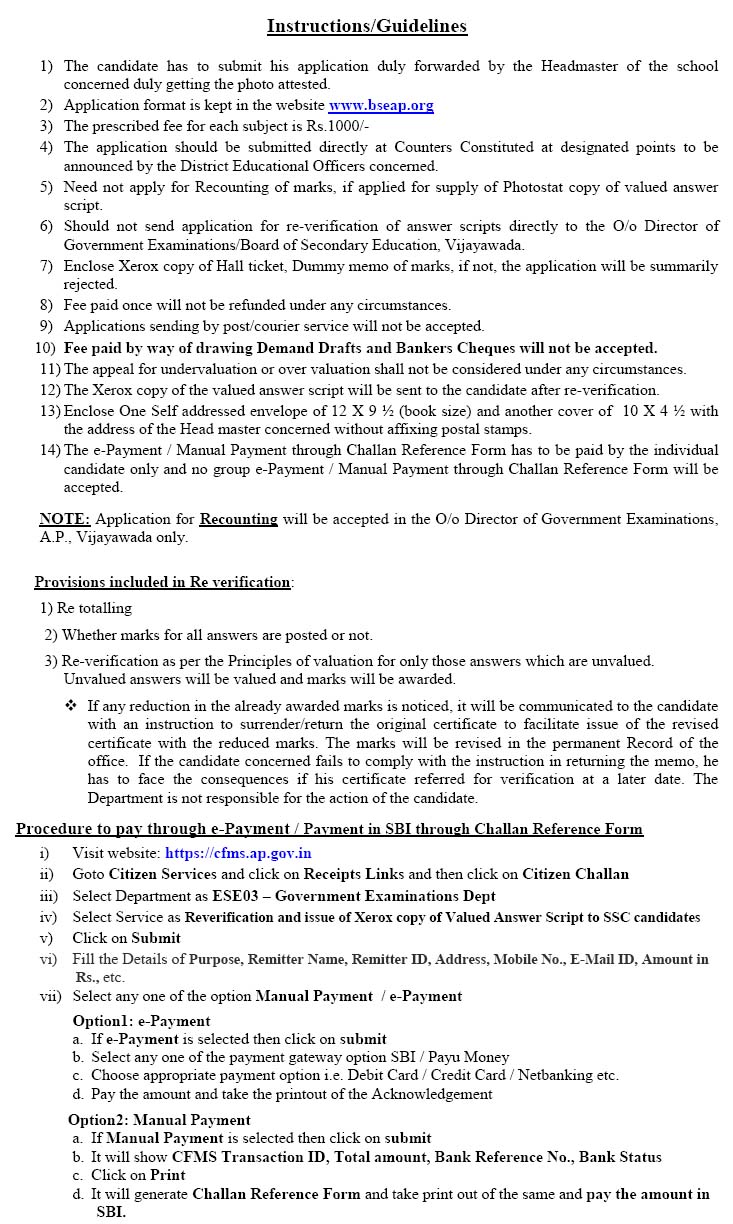**Detailed Caption for Website Screenshot**

The image captures a comprehensive list of instructions and guidelines from an official educational website, illustrating the procedural details for candidates. The header prominently reads "Instructions/Guidelines".

1. **Application Submission**: Candidates must submit their applications duly forwarded by their respective school headmasters, with photographs attested.
2. **Application Format**: The application format can be found on the website [www.bseap.org](http://www.bseap.org).
3. **Application Fee**: The prescribed fee for each subject is Rs.1000/-.
4. **Submission Procedure**: Applications should be submitted directly at counters constituted at designated points, as announced by the district educational officers.
5. **Recounting Applications**: Candidates need not apply for recounting of marks if they have already applied for a photostat copy of the valued answer script.
6. **Re-verification Application**: Applications for re-verification should not be sent directly to the Director of Government Examinations/Board of Secondary Education, Vijayawada.

Additional instructions include a note that applications for recounting will only be accepted at the office of the Director of Government Examinations, Vijayawada.

**Provisions Included in Re-verification**:
1. Reference totaling.
2. Verification that marks for all answers are posted.
3. Re-verification according to valuation principles for unvalied answers; unvalued answers will be marked and awarded accordingly.

**Footnote**: The website includes a footnote detailing the procedure for payment, either via e-payment or a manual payment process through SBI.

**Payment Procedure**:
1. **E-Payment/Manual Payment**:
    - Visit the website [https://cfms.ap.gov.in](https://cfms.ap.gov.in).
    - Navigate to "Citizen Services" and click on the "Receipts" links.
    - Click on "Citizen Chalan".
    - Follow additional steps for either e-payment or manual payment options.

This detailed description conveys the array of instructions and procedures captured in the screenshot, providing a clear guide for prospective candidates.